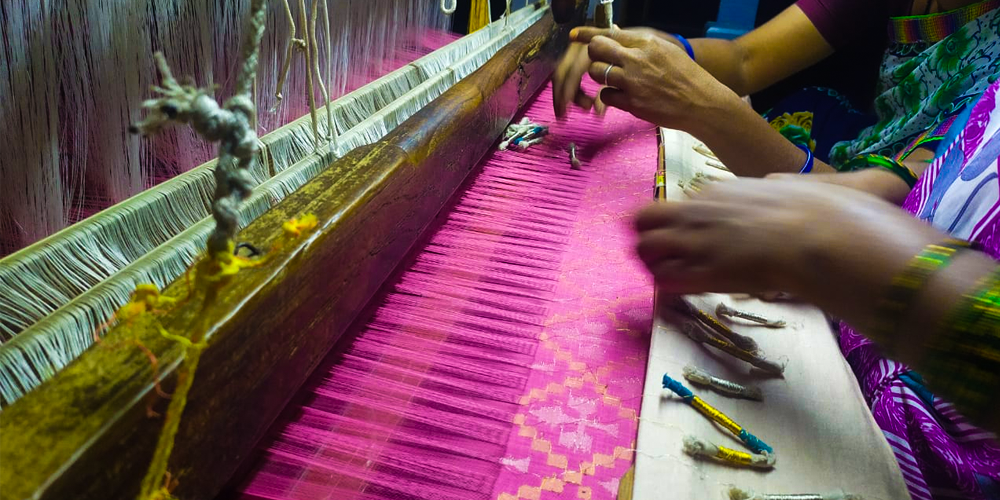In this indoor image, two women are deeply engrossed in the traditional craft of weaving, working on a colorful loom. They are adorned in vibrant, tribal-like attire featuring hues of purple, green, and an array of other striking colors. The scene is vibrant and detailed, with the women meticulously manipulating small thread pieces, some of which seem to be color samples, displayed on a white fabric in front of the loom.

The loom itself showcases predominantly pink and orange threads, interspersed with hints of gray, coming together beautifully in a complex pattern. Surrounding the loom are rows of thin white strings, organized and hanging down, attached to a long brown wooden bar that spans the length of the setup. The table they are working on is dominated by a long pink cloth adorned with intricate yellow and light pink patterns, adding another layer of visual richness to the scene. Various colored threads are scattered around, indicating the multitude of colors being used. Their hands move deftly over the loom, guiding the threads through the weaving process, creating a vibrant tapestry on the white fabric bordered by two wooden boards beneath the loom.